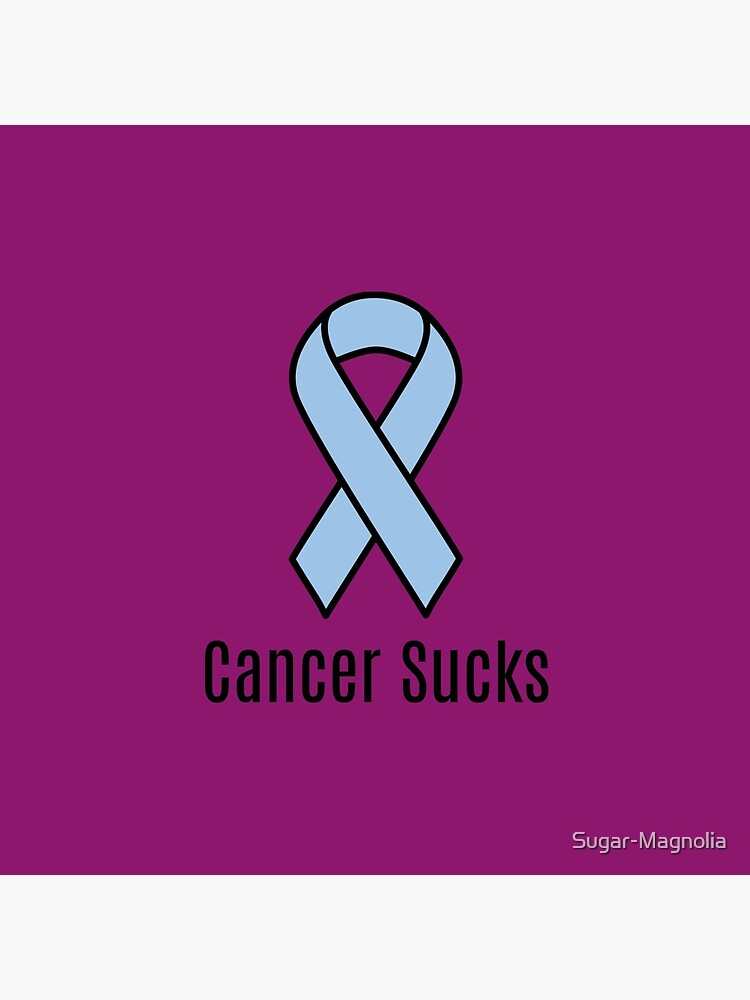The image is a precise digital artwork featuring a prominent cancer awareness ribbon. The background is a solid deep purple, reminiscent of Barney the Dinosaur’s hue. Centered on this background is a light blue ribbon, intricately folded to form a half infinity symbol, culminating in an X where the ends overlap. Directly beneath this ribbon, bold black text declares "Cancer Sucks." In the bottom right-hand corner, a small white watermark reads "Sugar Magnolia." The entire composition is simplistic yet impactful, with clean lines and a clear message.